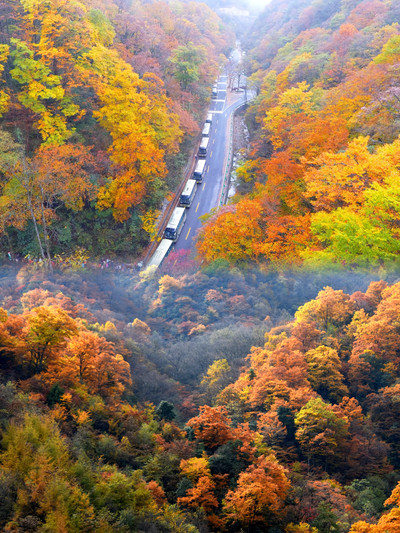This is an aerial photograph taken from a high vantage point, possibly by a drone or from atop a hill, capturing a breathtaking autumn landscape in North Georgia. The image is oriented in portrait style and prominently features a black-paved road with yellow center lines cutting through the picturesque scene. The road traverses the middle of the composition from the top to about halfway down, flanked on both sides by thick forests adorned in vibrant fall foliage, showcasing a stunning palette of orange, yellow, green, red, and hints of purple.

On the left-hand side of the road, a line of large, white buses or trucks travels toward the bottom of the photograph, their substantial size emphasizing their presence amidst the natural beauty. The road to the right appears empty, creating a contrast with the dense, colorful trees that extend to the edges of the image. The bottom half of the photograph is dominated by an even denser thicket of trees, further highlighting the richness of the autumnal colors that cloak the landscape.